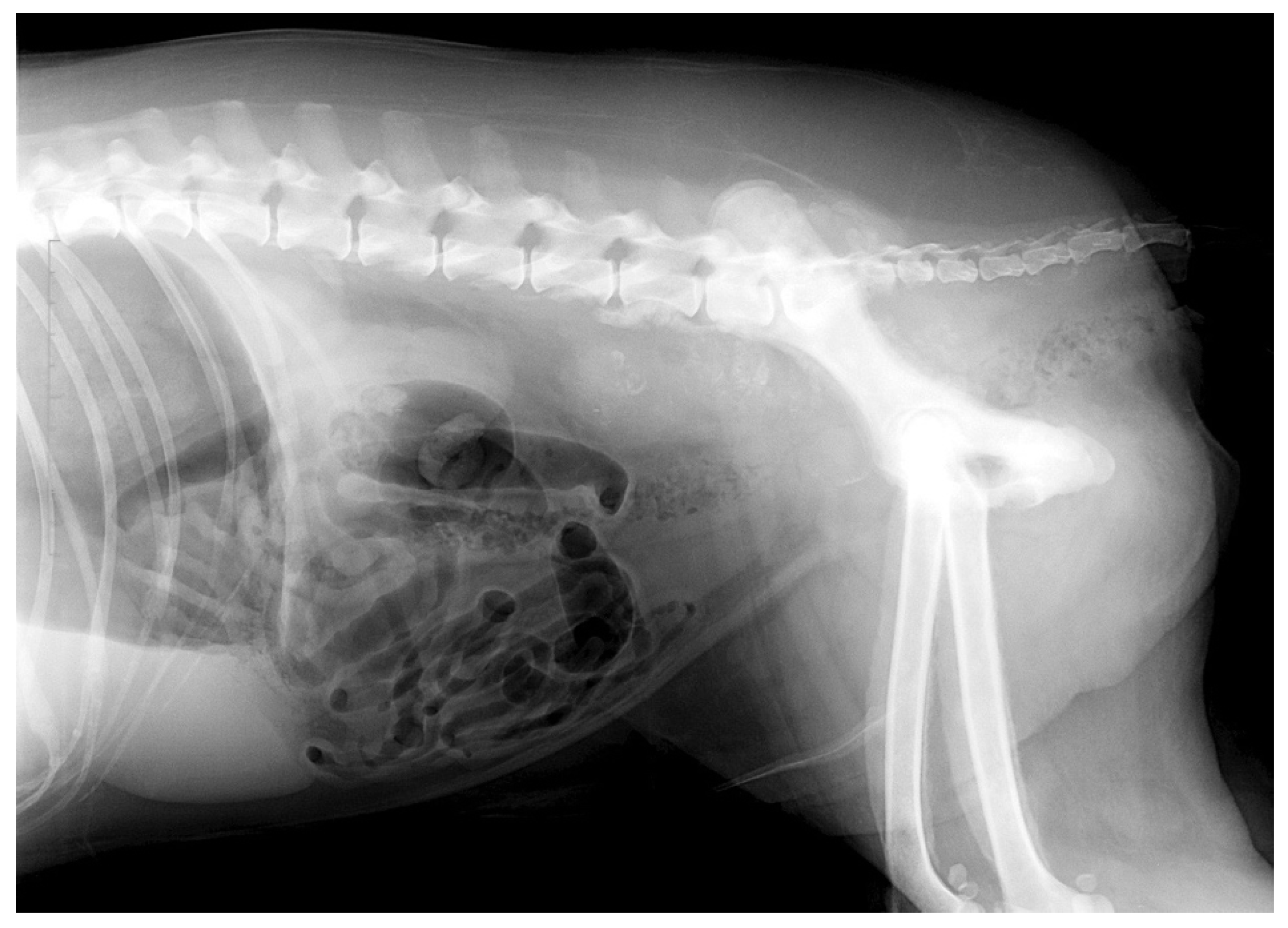This black and white X-ray image showcases the skeletal structure of what appears to be a dog. The prominent vertebrae run from the thick spine on the left, tapering off toward the right end of the image. The ribcage is distinctly visible, as are the pelvic bones and portions of the leg bones, with the pelvic bones appearing particularly dense and bright. Notably, the end of the tailbone is also visible. In the center of the image, within the stomach area, there's a conspicuous black mass, potentially indicating something the dog might have swallowed, though it's unclear due to the hazy, indistinct nature typical of X-ray images. These black formations suggest some sort of tangled or lodged material, contrasting sharply with the vivid white of the dense bones surrounding it.